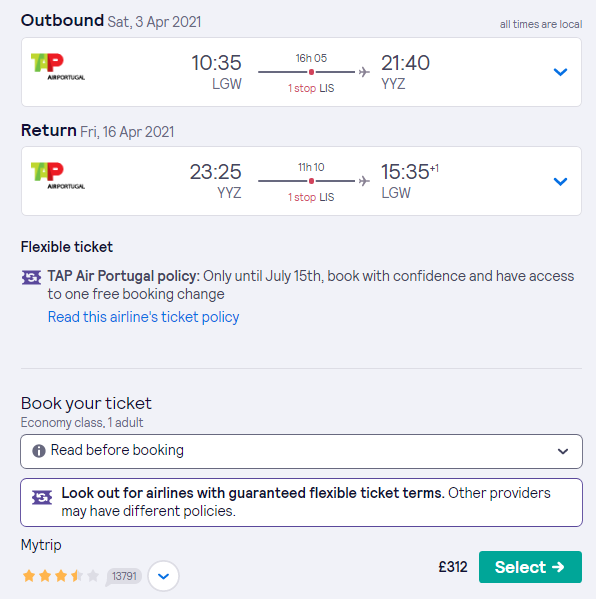### Detailed Caption:

This image displays information about outbound flights, specifically detailing an itinerary for a trip. It lists an outbound flight on Saturday, April 3, 2021. All times are indicated to be local. The first listing is for Air Portugal, with the flight departing at 10:35 and arriving at 21:40, resulting in a total journey time of 61 hours and 5 minutes from London Gatwick (LGW) to Toronto Pearson (YYZ), including a stopover in Lisbon (LIS).

The return flight is scheduled for Friday, April 16, 2021, also with Air Portugal. The flight departs at 23:25 from Toronto Pearson (YYZ) and arrives at London Gatwick (LGW) at 15:35, taking 11 hours and 10 minutes, with a stopover in Lisbon (LIS).

Underneath these details, there is a note regarding flexible tickets, mentioning TAP Air Portugal's policy. It states that bookings made until July 15 allow for "book with confidence" and include one free book and change. A clickable link is available to read the airline's ticket policy.

Following this information is a section labeled "Book your ticket" in which the economy class fare for one adult is displayed. There are two drop-down boxes: the first reads "Read before booking," and the second advises to "Look out for airlines with guaranteed flexible ticket terms," while indicating that other providers may have varying policies.

At the bottom of the screen, there is an option labeled "My Trip," which has a rating of three and a half stars based on 13,790 reviews. The listed price for the trip is 312 euros, accompanied by a button to select this option.